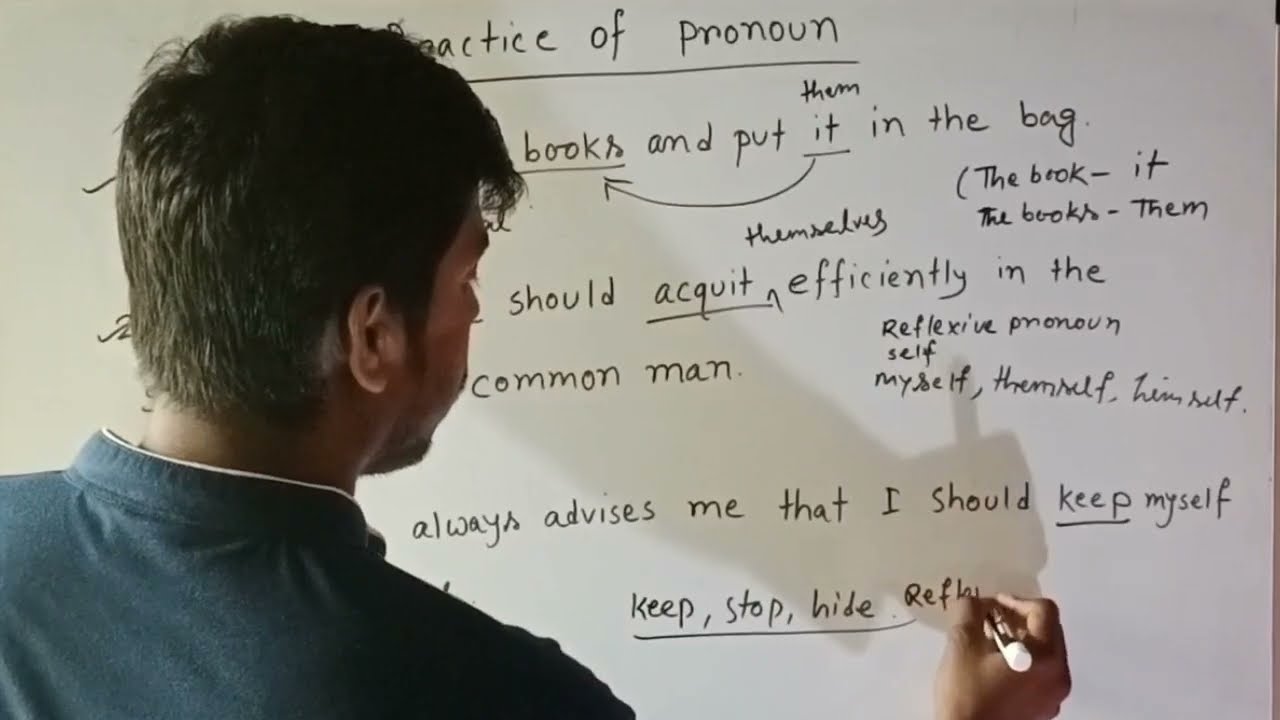The photograph captures a man, likely Indian, with dark skin and short hair, writing on a whiteboard using a black dry-erase marker. The image focuses on his upper body, showing him from the shoulders up, with his back to the camera and his right hand holding the marker. He is dressed in a dark gray shirt, which appears to be a polo.

The whiteboard, occupying the right side of the image, contains a detailed grammar lesson. At the top, the heading "Practice of Pronoun" is underlined. Below, various sentence fragments and grammar notes are scattered across the board. Phrases such as "books and put them or it in the bag" and "the book - it, the books - them" can be seen, alongside more complex sentences like "should acquit themselves efficiently in the common man."

There are also notes on reflexive pronouns including terms like "self," "myself," "themself," and "himself," with the advisory note "always advise me that I should keep myself," where "keep" is underlined and followed by "keep, stop, hide." Additionally, the partially written word "reflect" or a similar word beginning with "R-E-F" is visible.

A shadow of the man’s arm and pen casts diagonally across the whiteboard, suggesting that the light source is coming from the lower right. The detailed text on the board and the specific positioning of the man contribute to an instructional and educational setting focused on grammar practice.